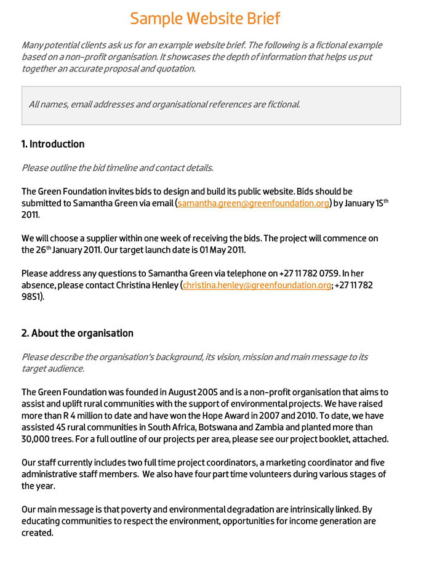Image Description: The image displays a detailed document titled "Sample Website Brief," presented in a vertical rectangle format. The title "Sample Website Brief" is prominently highlighted in an eye-catching orange color.

The document is clearly sectioned to organize the information effectively. An introductory note informs viewers that many potential clients request an example of a website brief. It emphasizes that the content is fictional and based on a non-profit organization, illustrating the level of detail required to create an accurate proposal and quotation.

A shaded box within the document clearly states, "All names, email addresses, and organizational references are fictional."

The document is divided into two main sections. 

**Section One: Introduction**
- This section advises on outlining the bid timeline and providing contact details.
- It includes a subsection indicating that proposals should be submitted to a specific individual, "Samantha Green," via email, with the email address displayed in orange.
- Another subsection offers contact information for addressing any questions, listing another email for "Christina Henley."

**Section Two: About the Organization**
- This area requests a description of the organization's background, vision, mission, and main message to its target audience.
- It provides an example of what such a description might look like, complete with a fictional review.

The layout, color usage, and structured format of the document aim to guide potential clients through the necessary steps to provide comprehensive information for website briefings.